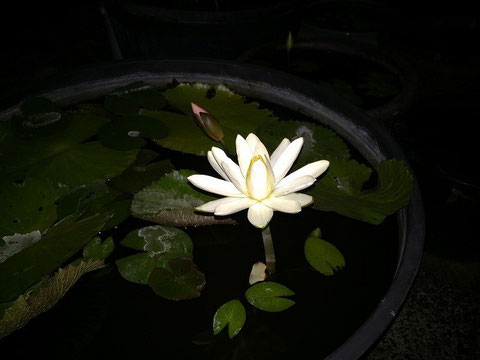The photograph centers on a striking white lily in full bloom, situated in a dark, likely watery environment. A brown pot holds the flower, but it's somewhat obscured by the murky surroundings. The lily stands out with its white petals, including one central petal that features a distinctive yellow border. The flower's gray stem elevates it above a mix of green foliage, contributing to a lush contrast against the dark backdrop. Some observers thought they saw lily pads or floating leaves scattered around, hinting at a possible aquatic setting. Overall, the image, although blurry, captures the serene beauty of the white lily against a dark and mysterious background with patches of green vegetation.